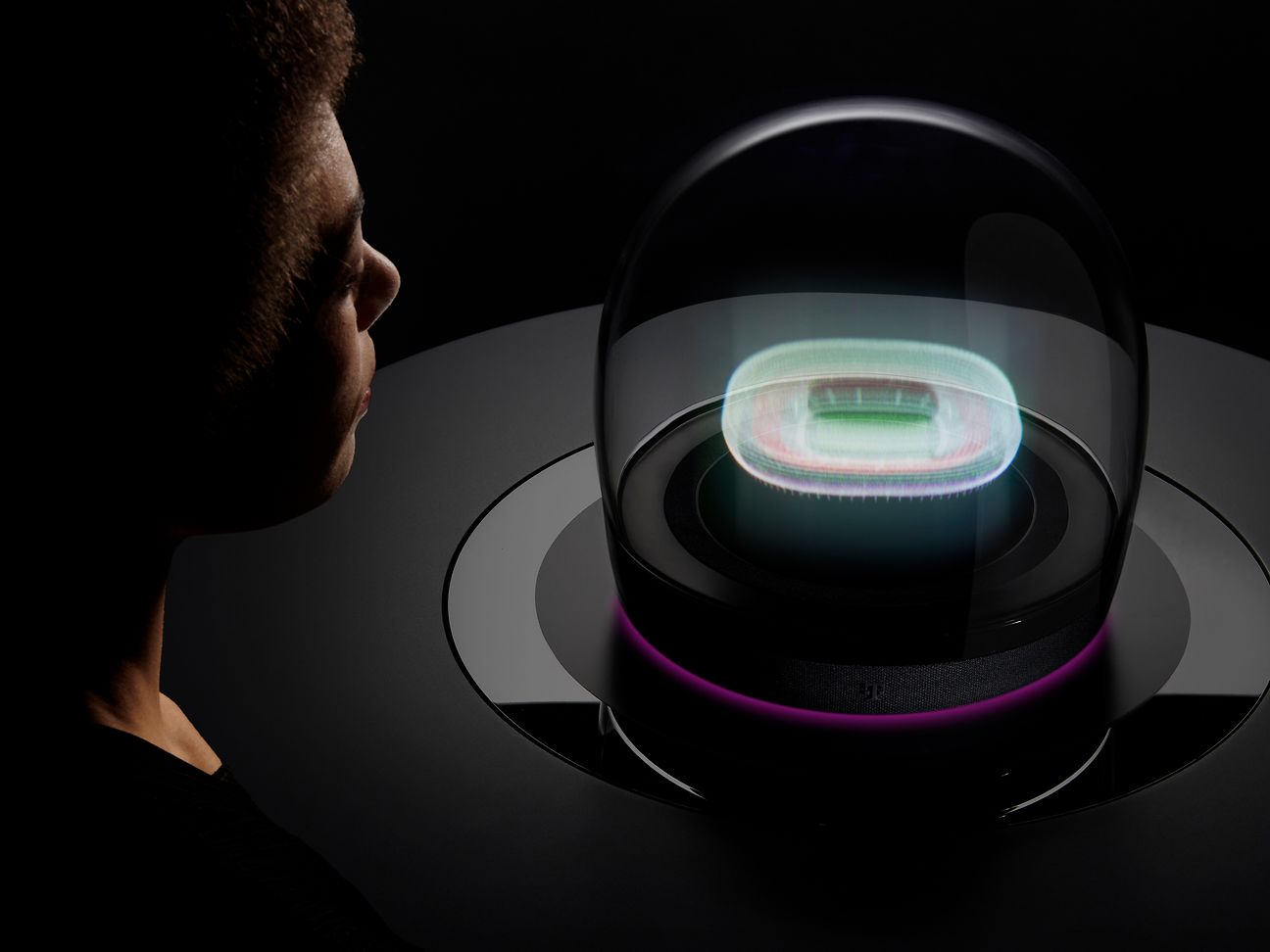In this striking futuristic image set against a completely black background, a dark-skinned woman with very curly hair, dressed in black, gazes intently at a holographic display. The hologram, housed within a transparent black dome, depicts an empty football stadium, brought to life in vivid three-dimensional light. Situated on a matte black table, the dome is framed by a distinctive shiny ring that resembles the shape and size of a Roomba. From beneath the hologram, a gradient of purple and pinkish-magenta light emanates, casting an otherworldly glow that highlights the intricate details of the stadium. The image is captured from a top-down perspective, ensuring every detail is clear and immersive, bringing to life the blend of advanced technology and cinematic design.